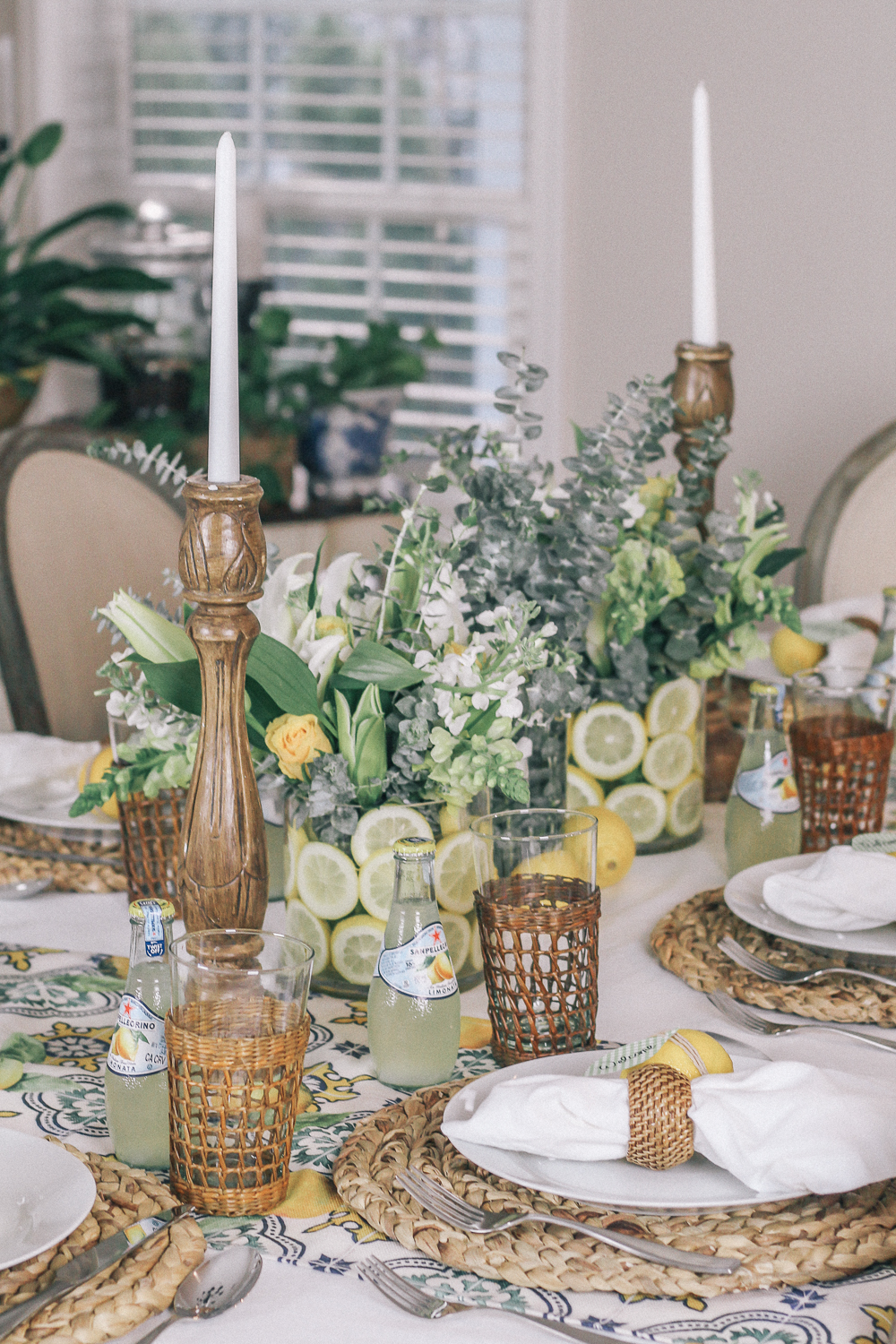The image showcases a beautifully set dining table that exudes a charming, rustic elegance. The table is adorned with a vividly patterned tablecloth featuring a palette of white, yellow, blue, and green. On top of this, wicker placemats crafted from woven knots of rope provide a textural contrast. At each place setting, there is a pristine white plate accompanied by a neatly folded napkin secured with a wicker napkin holder. The glasses, too, are encased in woven brown straw holders, and next to each glass is a bottle of Pellegrino lemon water.

The centerpiece of the table is particularly striking, consisting of clear glass vases filled with white and pale green flowers, interspersed with bits of eucalyptus leaves. The vases are creatively embellished with lemon slices pressed against the glass, adding a touch of freshness and color. Flanking the centerpieces are two elegant candlesticks with metal holders featuring intricate designs, each cradling a white tapered candle.

The table setting is completed with a couple of whole lemons placed casually on the table, enhancing the citrus theme. Surrounding the table are white chairs, and in the background, a window with open blinds allows natural light to filter into the room. Green potted plants sit on a nearby table by the window, adding a touch of nature to the serene ambience of the dining area.